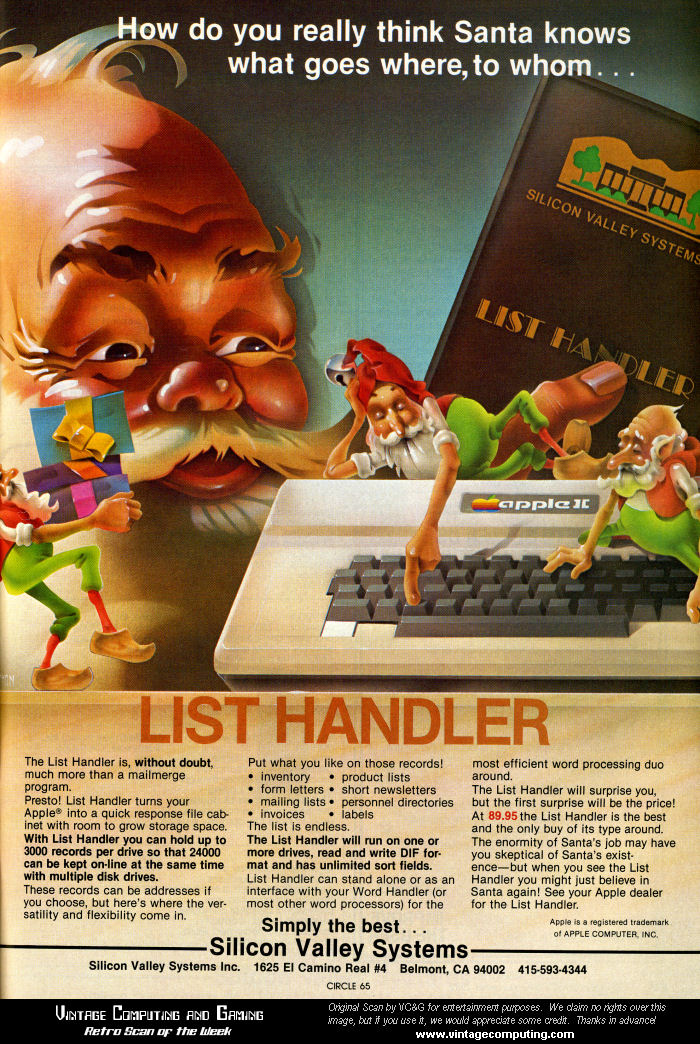In the image, there is a vintage advertisement with a predominantly green background. At the top, it features the text in white letters, "How do you really think Santa knows what goes where to whom?" The centerpiece depicts Santa Claus with a white beard, mustache, and rosy cheeks, looking delightedly ahead. His eyes, framed by wrinkles, impart a cheerful expression. 

Santa is interacting with three elves, who are all engaging with an Apple II keyboard. One elf is laying down and punching the keys, another is bracing himself on the keyboard, and the third elf, who is near Santa and whose face is not visible, is carrying a box of presents. The keyboard is prominently branded as an Apple II.

Beneath Santa and the elves, the large orange block letters spell out "List Handler," followed by further descriptive text about the product, emphasizing its utility as a comprehensive data management system that can handle up to 24,000 records with multiple disk drives. The text extols its versatility for uses ranging from mailing lists to inventory management. At the bottom, it states, "Simply the best: Silicon Valley Systems," along with the company's address and contact information in Belmont, California.